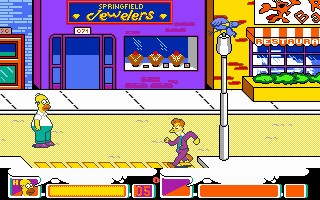In this vivid cartoon scene from "The Simpsons," Homer Simpson is standing on a yellow-toned road, donning his signature ensemble of blue pants and a white t-shirt. The setting includes a detailed sidewalk, which is colored white. On this sidewalk, a man dressed in a vibrant purple outfit appears to be briskly walking past Homer. The backdrop features several buildings: Springfield Jewelers, characterized by its purple facade, a neighboring blue building, and a yellow building suspected to be a restaurant. A white street light stands nearby, contributing to the urban atmosphere. Homer's expression conveys a sense of perplexity, adding to the narrative depth of the image. The scene is framed with yellow and orange elements at the bottom, resembling game scores, further suggesting that this visual is part of a gaming context.